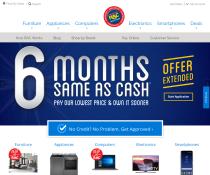The captured image depicts a website with a white background, although it appears to be of low quality and very blurry. At the top left of the page are two gray buttons, while the top right has two additional buttons, likely for login purposes. In the center of the top section, there is a red circle with a blue circle inside, presumably the website's logo. Flanking the logo on both sides are three clickable blue text links, though they are too blurred to decipher.

Dominating the central portion of the website is a large blue rectangular area. At the top of this rectangle is a gray strip containing dark gray text, which is also too blurry to read clearly. Prominently displayed within the middle of the blue rectangle is large gray text that states, "Six months same as cash. Pay our low price and own it sooner." On the right side of this message is yellow text reading, "Offer extended."

Beneath the blue rectangle is a lighter blue rectangular section with white text and a check mark, though the specific wording remains unclear due to the blurriness. 

At the bottom of the website, there are five images: a living room, a printer, a laptop, a TV, and what appears to be a cell phone. Above these images is blue text listing categories that likely read, "Furniture, Appliances, Computers, Electronics," and possibly "Smartphones."